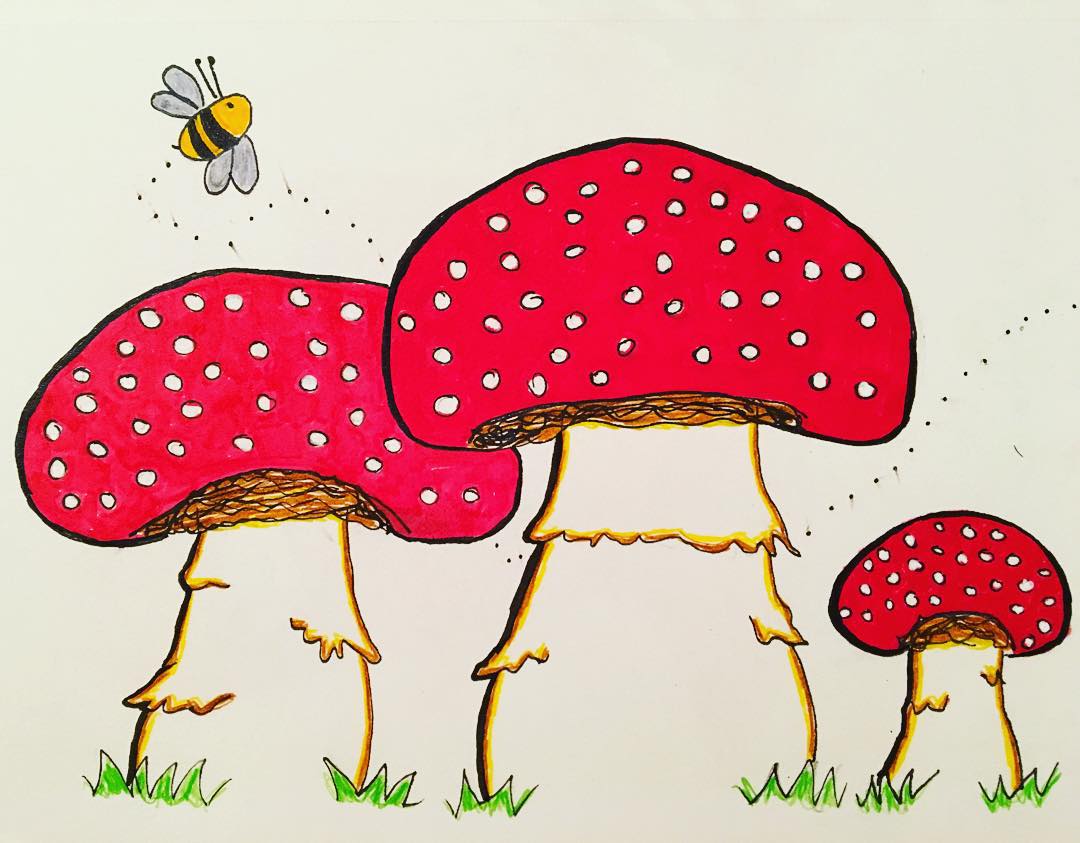This detailed illustration vividly depicts a serene forest clearing dominated by three large, vibrant red mushrooms adorned with white spots on their caps. The mushrooms feature sturdy, thick white stems rooted firmly into the forest floor, with tufts of green grass sprouting around their bases. In the scene, two mushrooms are prominently positioned in the foreground, while a third stands subtly in the background, adding depth to the composition.

In addition to the lush greenery, the image highlights a bee hovering near the mushroom trio. The bee, characterized by its four delicate wings (two on each side), black antennae, tiny single eye, and two black stripes along its yellow body, is seen in motion, trailing a dotted path that weaves from the center right of the frame, behind the mushrooms, and upward into the sky. The bee’s lively presence injects a sense of movement and life into this tranquil woodland setting.